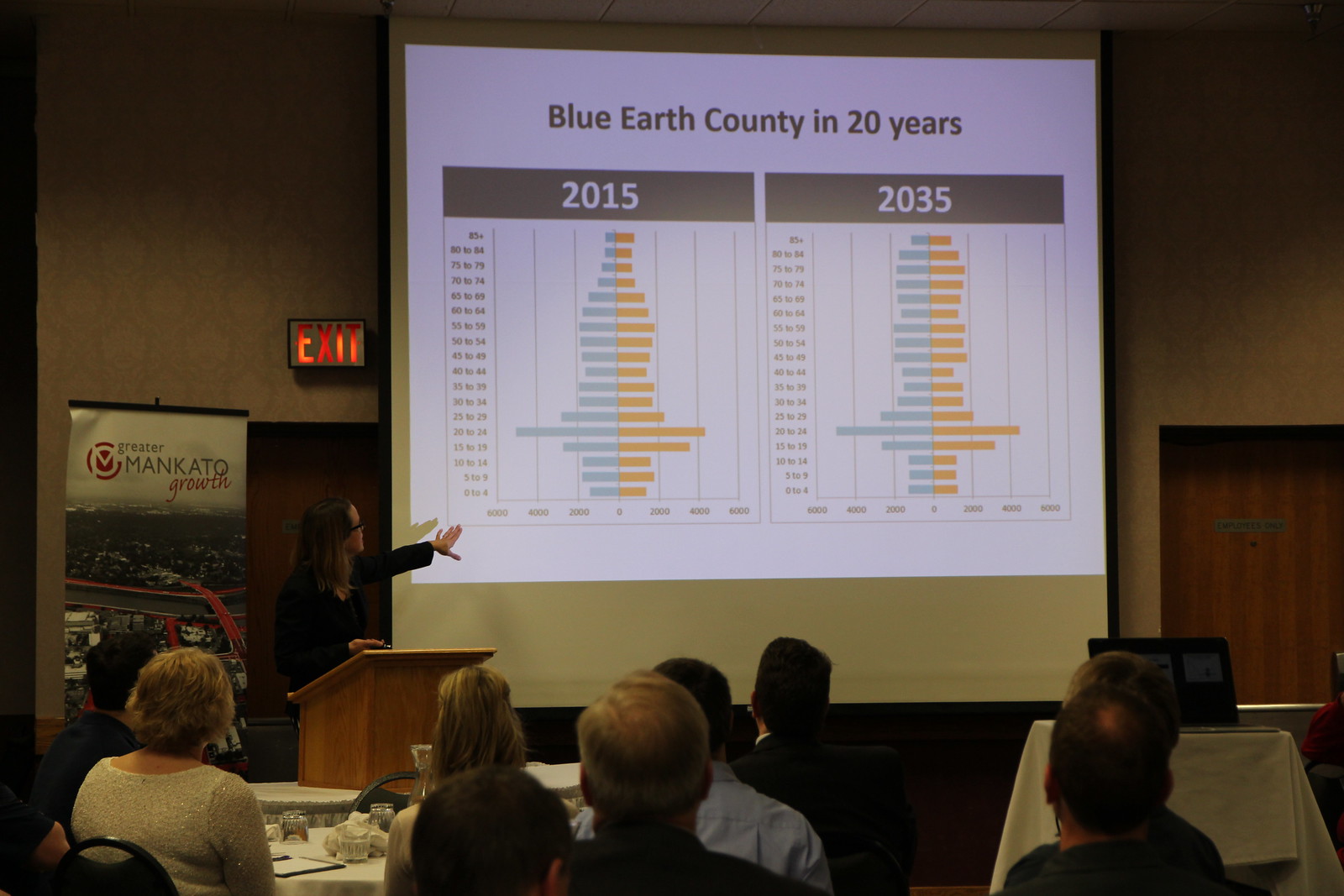A woman, who appears to be Caucasian with shoulder-length blondish-brown hair and black glasses, stands at a podium in front of a projection screen delivering a presentation. She is wearing a long-sleeve shirt and is pointing to the screen with her left hand. The screen displays the title "Blue Earth County in 20 Years," with two columns beneath it: the left column labeled "2015" and the right column labeled "2035," each accompanied by graphs that feature lighter blue and orange colors respectively. The presentation takes place in a cream-colored room. On the left side of the screen, a banner reads "Greater Mankato Growth," suggesting the focus is on the town of Mankato. An exit sign is visible to the left of the screen, above a brown door, with another matching door on the far right. In the foreground, attendees are seated at tables with their backs to the viewer, including several men and women, all attentively facing the speaker.